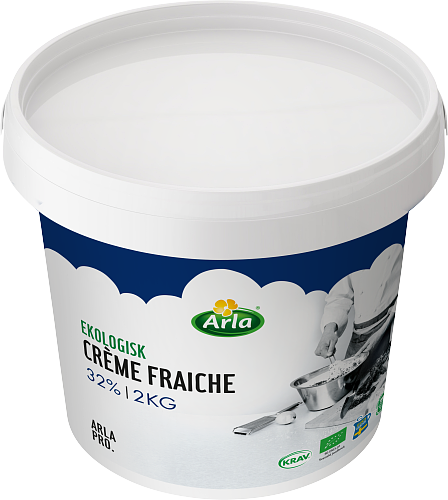The image depicts a container of crème fraîche from the brand Arla. The container features a predominantly white base, with a design that includes white fluffy clouds towards the top, giving way to a blue strip. The white lid is detachable. Centrally located is the Arla logo, consisting of a green oval with white 'Arla' text, topped with a yellow flower. The text on the container includes "Ecologique" in green, "crème fraîche" in black, and "32% 12 kg" in blue. Below, "Arla Pro" is printed in black text. There is an image of a chef, with only the torso visible, cooking in a silver pan with silver utensils nearby and an egg placed on the counter beneath the pan. Additional logos are present at the bottom right, below the cooking image, representing the product's safety and other attributes.